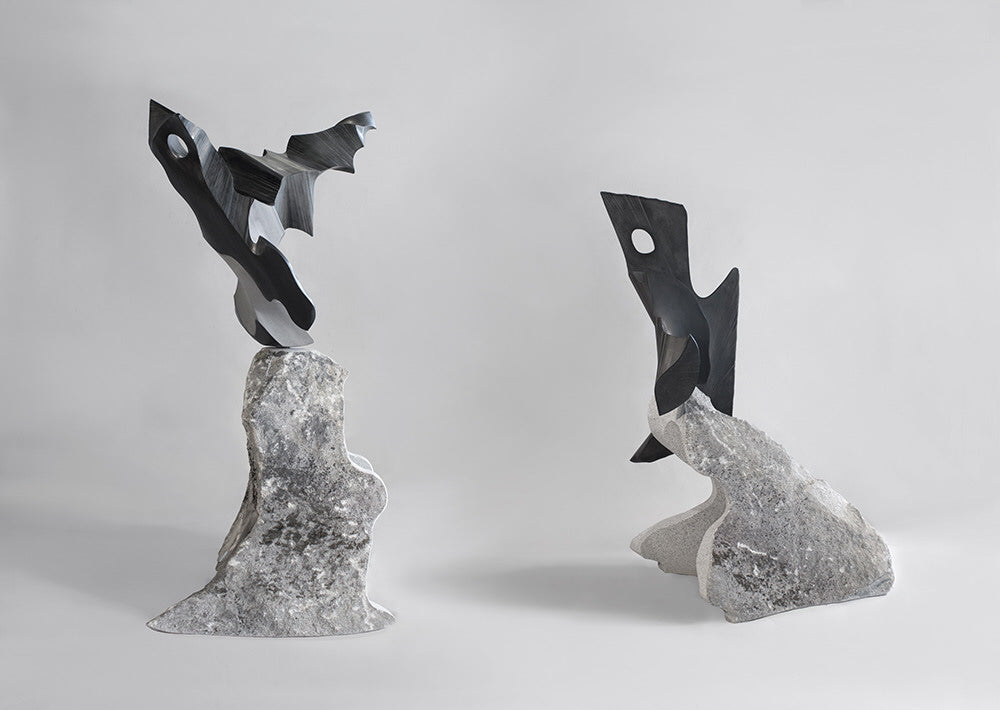The image showcases two abstract sculptures set against a nondescript background in a black and white photograph. Both sculptures have bases that appear to be crafted from a whitish-gray stone or mineral material, lending a crystalline texture to their forms. From a side view, the left sculpture features a tall, pointed black object that protrudes upwards, resembling an abstract form akin to a penguin with a wing extending to the right and a distinct hole near the top, suggestive of an eye. The sculpture on the right is similarly abstract but slightly smaller with a unique shape; it also has a hole at the top and lacks the pronounced wing-like extension from this perspective. Shadows cast from the right side of the image add depth and dimension, enhancing the enigmatic and contemplative quality of the artworks.